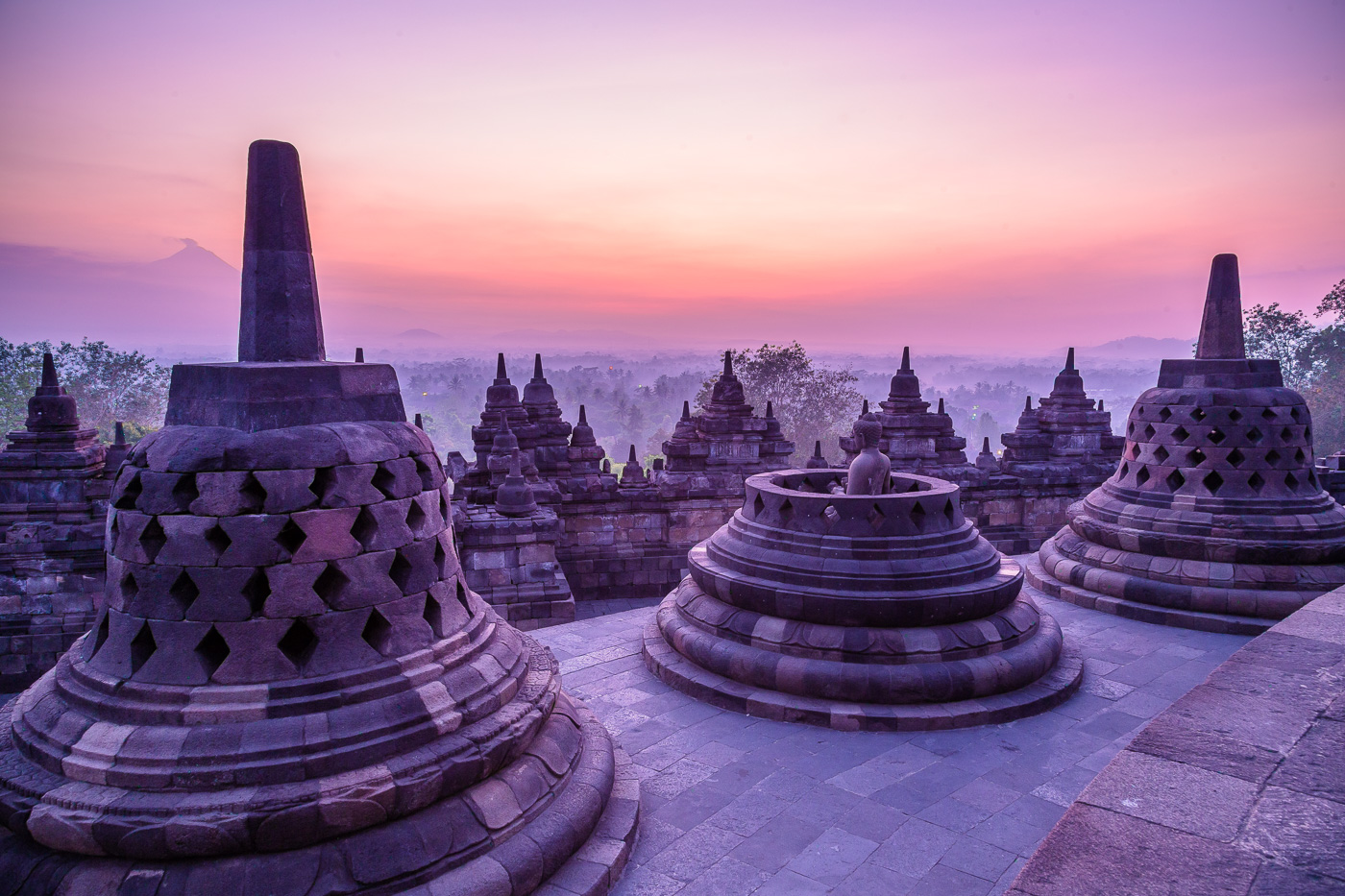This image captures a serene dusk scene from the rooftop of a temple, dominated by hues of purple, pink, and amber as the sun sets. The sky is a gradient of light purple, pink, orange, and beige, giving a tranquil backdrop. The foreground features several stone domed structures resembling bells, with one on the left, one near the center-right, and another on the far right. These domes are assembled from blocks, with some topped by spiked adornments. The central dome is open at the top and contains a stone figure looking towards the horizon. In the distance, smaller similar structures line the edge of the building, set against a backdrop of a vast valley dotted with numerous trees, accentuating the high vantage point of the temple.